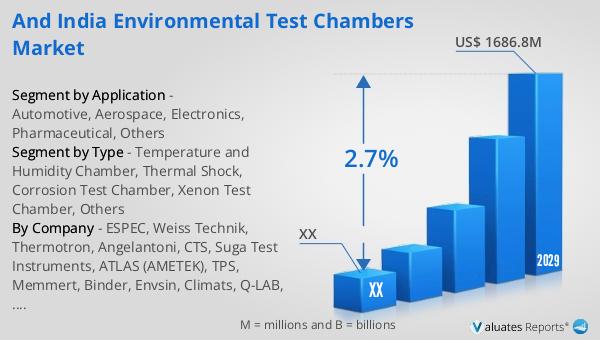The image is a detailed infographic slide focused on the financial trends in India's Environmental Test Chambers Market. At the top, the title "India Environmental Test Chambers Market" is prominently displayed in blue. The primary visual feature is a blue, 3D bar graph on the right side that illustrates a U.S. revenue increase from earlier years leading up to 2029, where the highest value reaches USD 1,686.8 million with a 2.7% growth indicated by an upward arrow. The left side of the image has various text segments in black detailing market breakdowns: "Segment by Application" which includes categories like automotive, aerospace, electronics, pharmaceutical, and others; "Segment by Type" listing chamber types such as temperature and humidity chambers, thermal shock chambers, corrosion test chambers, xenon test chambers, and others; and "Segment by Company" highlighting leading companies such as SPEC, Weiss Technic, Thermotron, Angela and Tony, CTS, Suga Test Instruments, Atlas, Amatek, TPS, Memmert, Binder, Envision, Climax, and QLAB. At the bottom of the slide, annotations clarify that "M" stands for millions and "B" stands for billions. The data source is credited to Evaluates Reports.